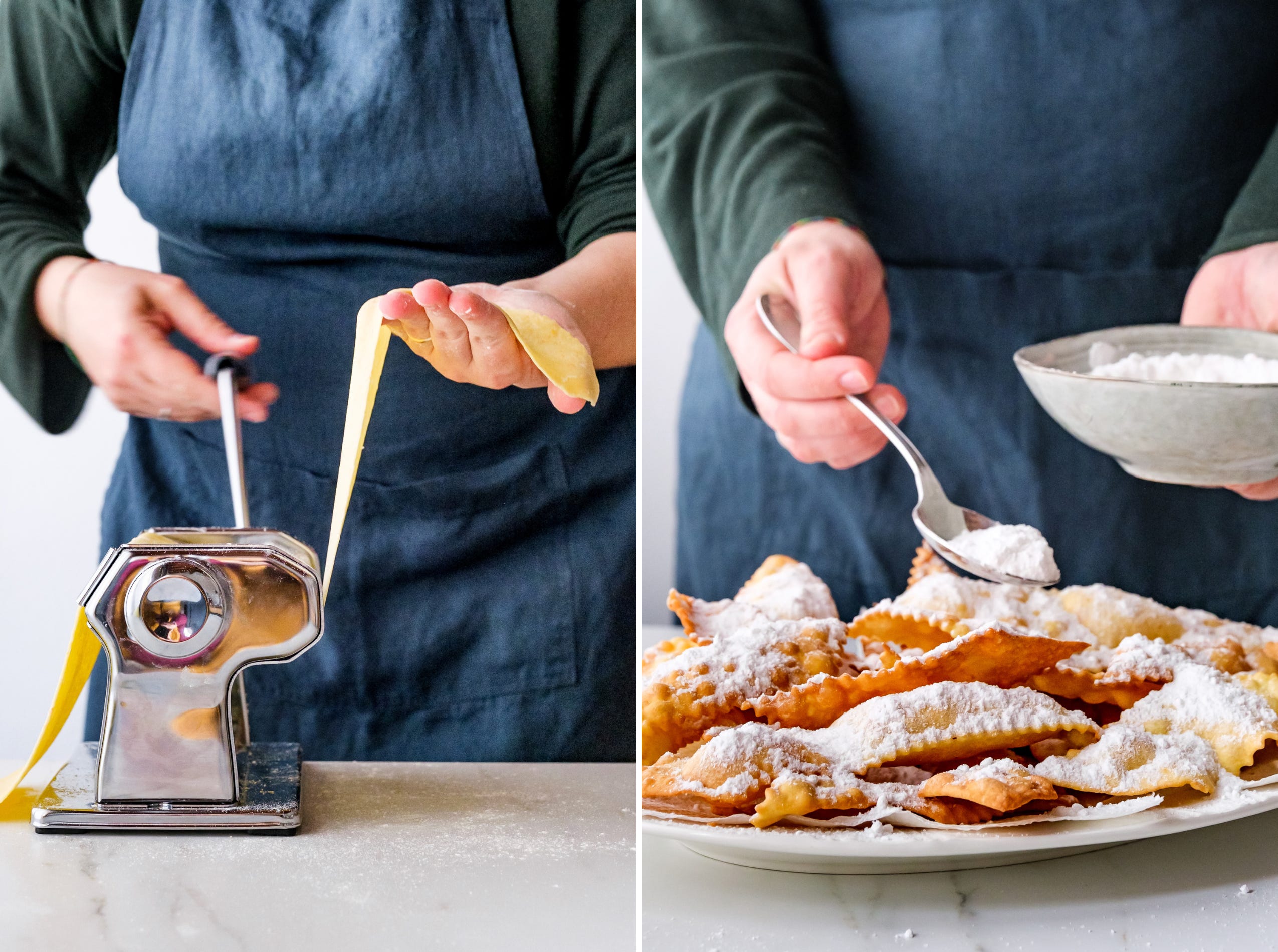In the first image, a person is seen wearing a long-sleeved black shirt with a blue apron over it. The viewpoint is from the abdomen down, focusing on their hands as they crank dough through a silver pasta machine on a pristine white surface. The machine feeds the dough in on one side and produces thin, even pasta on the other end.

In the second adjacent image, the same person is frying dough packets, possibly ravioli or a type of dessert. They're shown sprinkling powdered sugar over a plate of these golden-brown delights, which look crispy and perfectly fried.